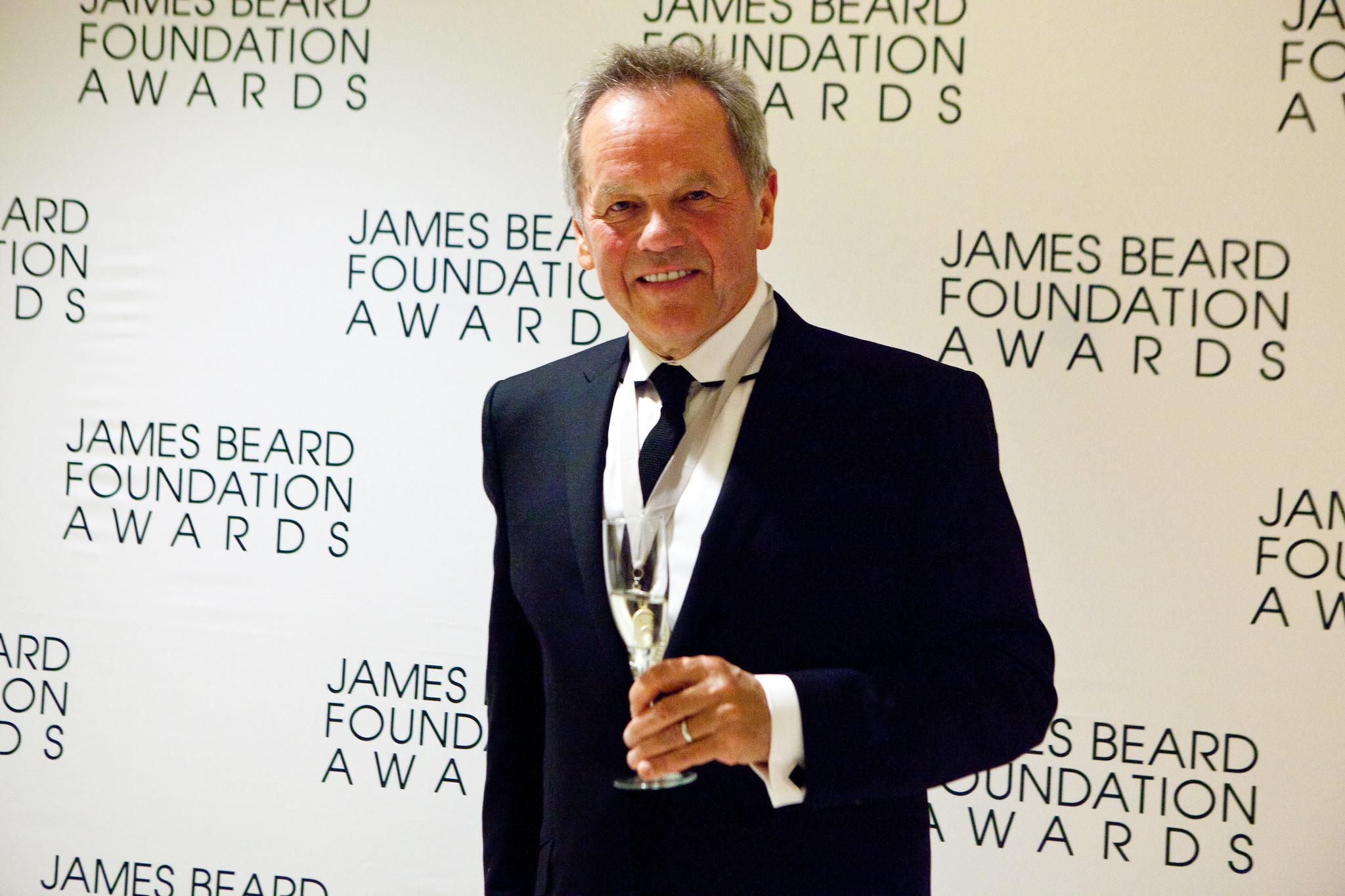The image depicts an older, famous white male, possibly a British or European chef, characterized by his salt-and-pepper thinning hair and tan skin. He is dressed in a dark, possibly navy blue or black suit jacket, paired with a white collared shirt and a black tie. A natural-colored lanyard hangs around his neck and a silver wedding band adorns his ring finger. The man is smiling warmly while holding a half-full champagne glass in his left hand. He is standing in front of a white ivory backdrop with the words “James Beard Foundation Awards” written in dark lettering. The rectangular photo is positioned horizontally.